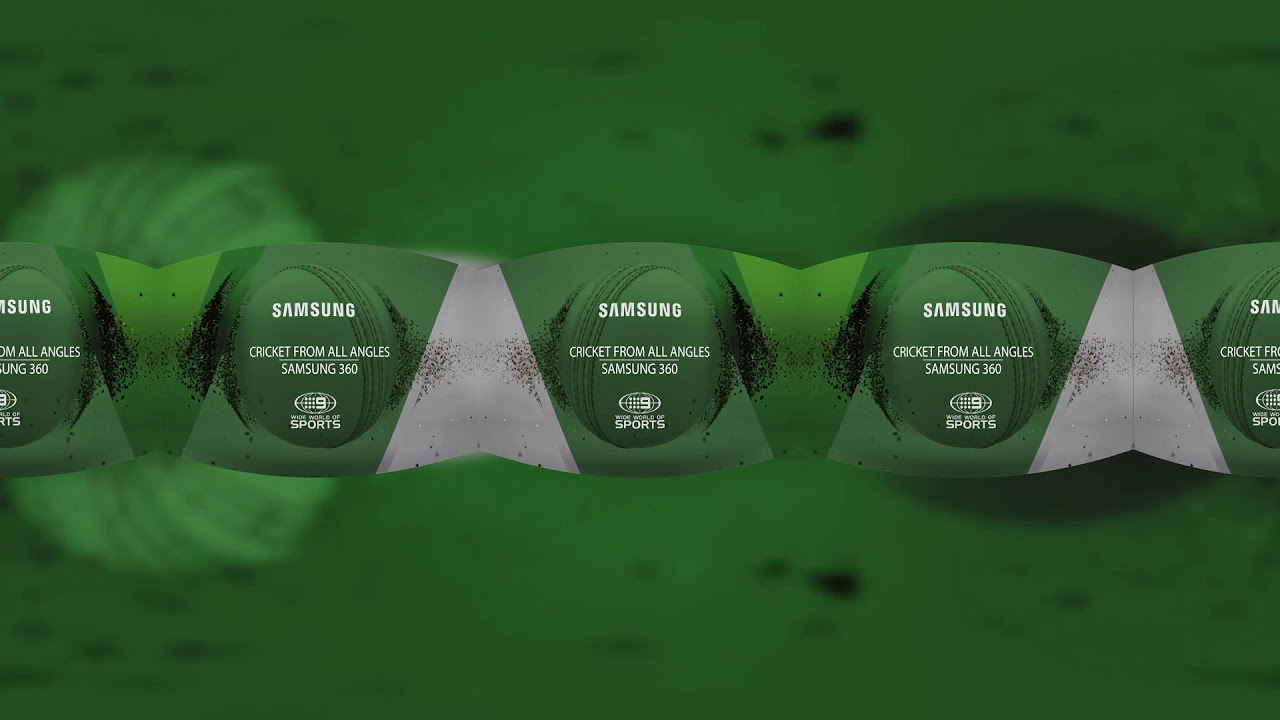This image appears to be an advertisement for Samsung, specifically promoting a Samsung 360 cricket viewing feature. The composition is primarily a wide horizontal rectangle dominated by a dark green background with scattered black splotches for contrast. Centrally positioned is a horizontally running cylindrical shape, segmented repeatedly into five distinct sections that resemble a snake-like form with undulating bulges and narrows. Each segment comprises a dark green bulge transitioning smoothly to a lighter green narrow. Across the dark green bulges of these segments, the text "Samsung, cricket from all angles, Samsung 360" is prominently displayed. Additionally, a small trademark symbol associated with World of Sports is visible. The cylindrical shape, with its alternation of tones and repeating segments featuring white and green triangles along with circular areas containing the key text, creates a dynamic visual effect reminiscent of a cricket ball seamlessly integrated with the vibrant green field suggested in the background.